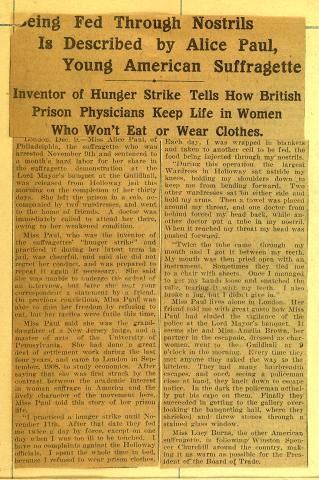This image is a photograph of a vintage newspaper article, visibly aged with a yellowish-brown hue, indicating its antiquity. The thinness of the paper is evident as the yellow lined background paper beneath it is visible through the article. The headline, prominently displayed in black text, reads, "Being Fed Through Nostrils is described by Alice Paul, young American suffragette." It goes on to state, "Inventor of Hunger Strike tells how British prison physicians keep life in women who won't eat or wear clothes." The newspaper article, which appears to have been cut out and possibly pasted onto the lighter yellow background, is comprised of two columns of faded text. The upper section of the headline is slightly torn, particularly the 'B' in "Being," suggesting some damage or detachment over time. The image does not contain any photos, focusing purely on the textual content, and might be a cut-out intended for a scrapbook.